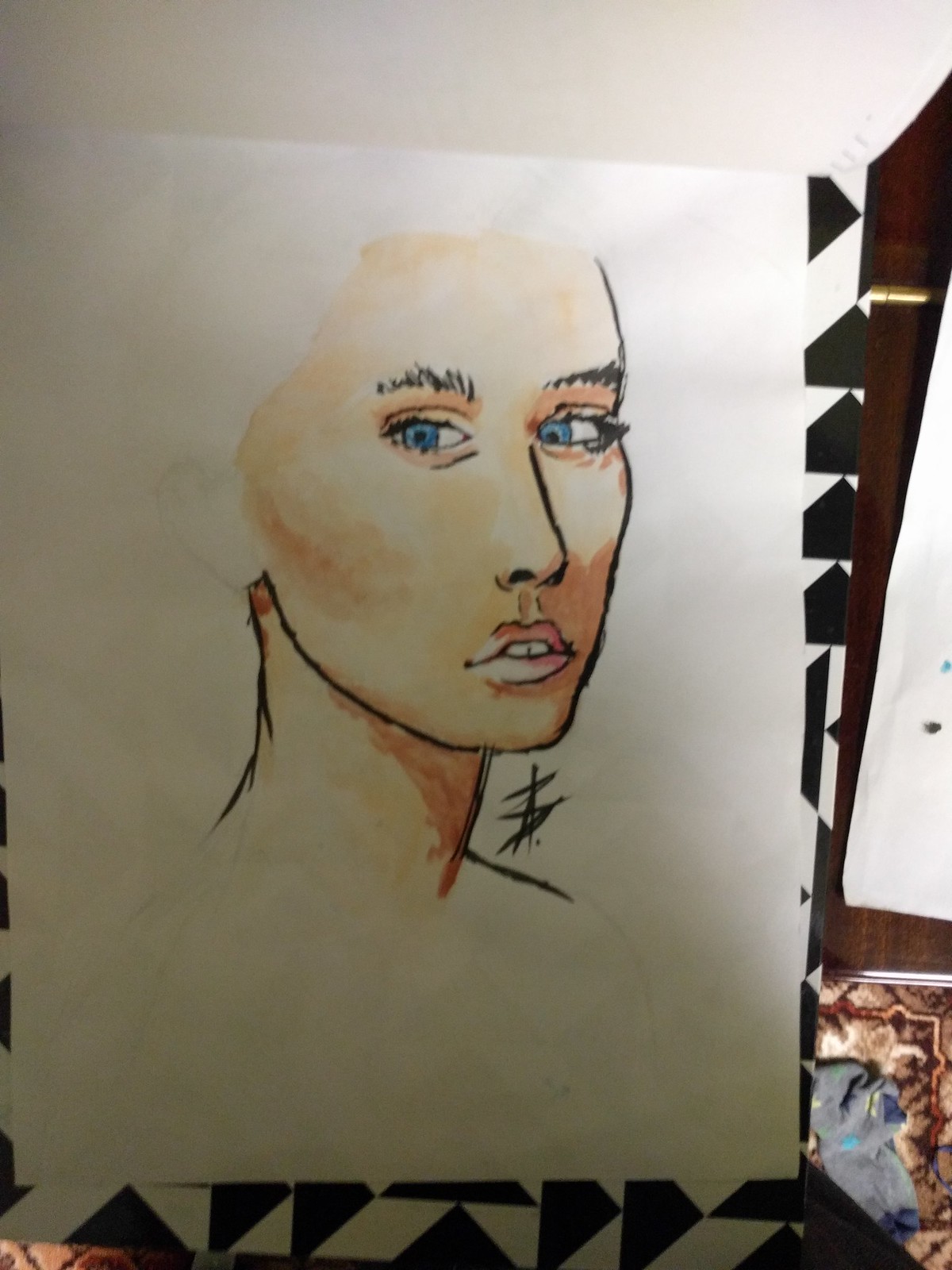This detailed photograph captures a hand-drawn portrait of a young woman on an A4 sheet of paper, possibly created with a combination of black pen or ink and watercolor. The artwork depicts the woman's face from the forehead down to her neck, highlighting her prominent eyebrows, blue eyes, and pink lips. Her long face is complemented by a white complexion and subtle orange shading, with blush visible on her cheeks and orange eyeshadow above her blue eyes. The piece appears slightly unfinished, with her hair and ears traced but not colored in.

The woman is depicted looking slightly to her left, with a hint of a smile showing two teeth. The drawing is centered on the paper, with the rest left mostly blank. Below her chin, there is a scribbled section, and an artist's signature is visible nearby. The portrait is bordered by abstract geometric patterns, featuring black and brown on the side and a blue and brownish-red abstract design in the bottom right corner. The photograph of the drawing was taken in low light, and some dirty laundry can be seen in the bottom right of the image, indicating the casual setting in which the art was captured.